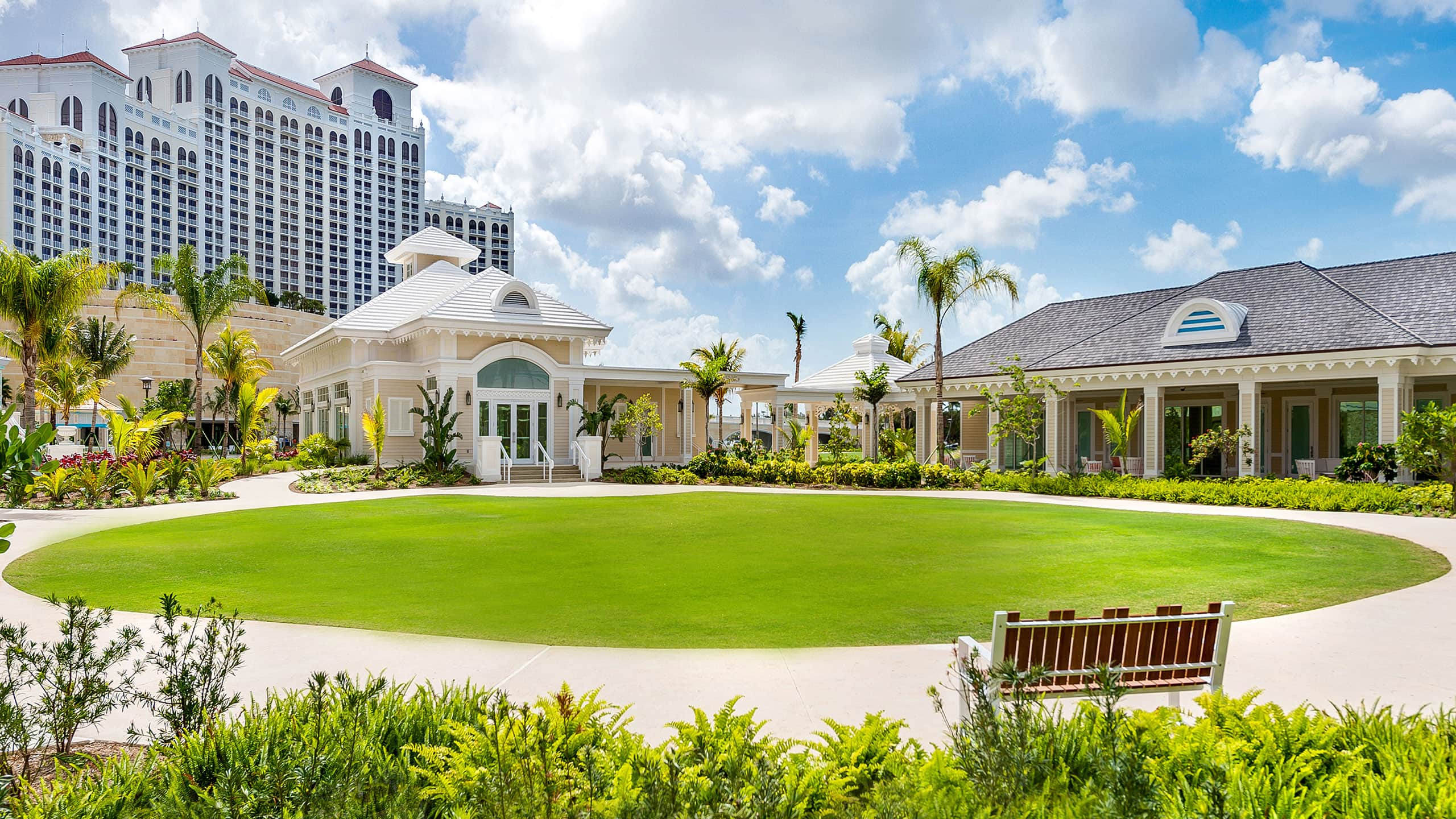The image showcases a luxurious outdoor area that exudes the charm of a high-end hotel or an opulent residence. Dominating the foreground is a perfect circle of lime green grass, its blades shimmering in the sunlight. Encircling this lush patch is a pristine white cement sidewalk. Nestled at the bottom right of the scene is a white-framed bench with wooden slats, facing towards the circular lawn and away from the viewer.

The architectural landscape includes multiple structures: to the right, a large, sprawling house with a gray roof, surrounded by lush plants. On the left side, there's a housing unit with a distinctive white-topped gazebo nearby, boasting a taller ceiling. Additionally, there is a substantial apartment building positioned further back, characterized by numerous windows and balconies, giving a sense of grandeur akin to a hotel resort.

The setting is further enhanced by a meticulously maintained garden and the presence of palm trees, adding a touch of tropical elegance. The daylit sky is a bright blue, accented with scattered clouds. The color palette within the image spans from blues and whites to earthy tones of tan, beige, and brown, punctuated by shades of green from the flora, and occasional hints of silver and black. The photograph appears to be taken from behind the bench, offering a comprehensive view that captures the idyllic and serene atmosphere of this lavish outdoor space.